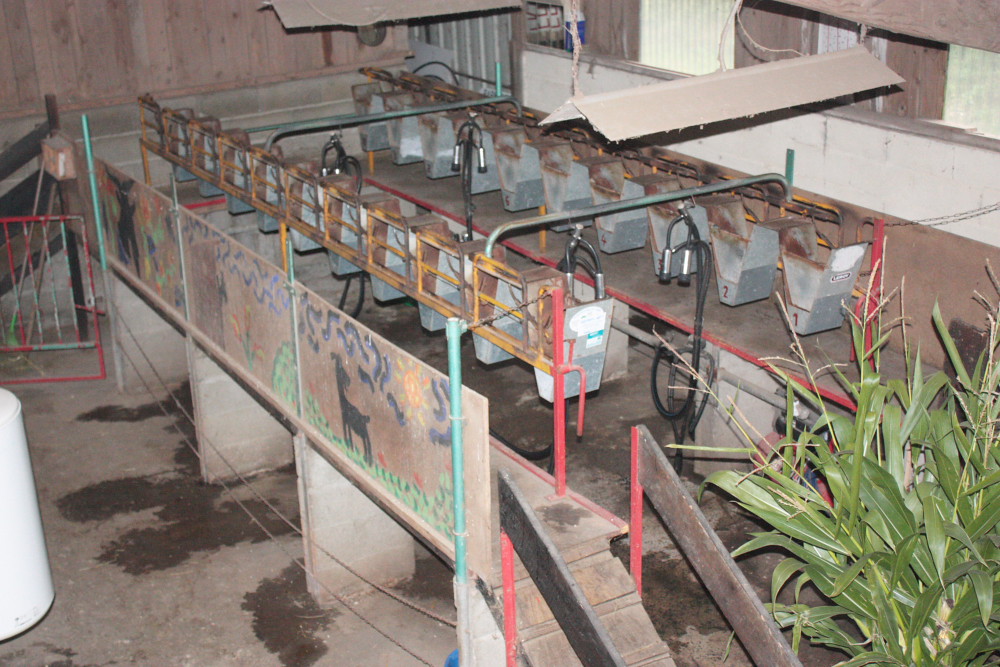The photograph depicts a dilapidated, rust-colored building exterior, appearing to be part of an old factory or animal care facility. The stained brown concrete ground is adorned with numerous triangle-shaped silver metal buckets, possibly part of an irrigation system, some positioned along the front ledge of the building. A wooden ramp enters the scene from the bottom right, beside which a small green plant with young offshoots can be seen. To the left, a large white cylindrical holding tank partially exits the frame. The fence at the back features peeling paint in shades of red and bluish-green. There are three enclosure openings or outcodes beneath the building, next to a fence topped with a mosaic of animals set on a grassy field under a shining sun. Painted pictures of animals adorn the building, suggesting its use for animal-related activities such as feeding or milking. Metal components, some painted red or yellow and showing signs of rust, are visible, along with a red-numbered feeder system that is arranged from right to left with numbers ascending from 1 to 4. Overhead lighting fixtures can be seen adding illumination to the scene.